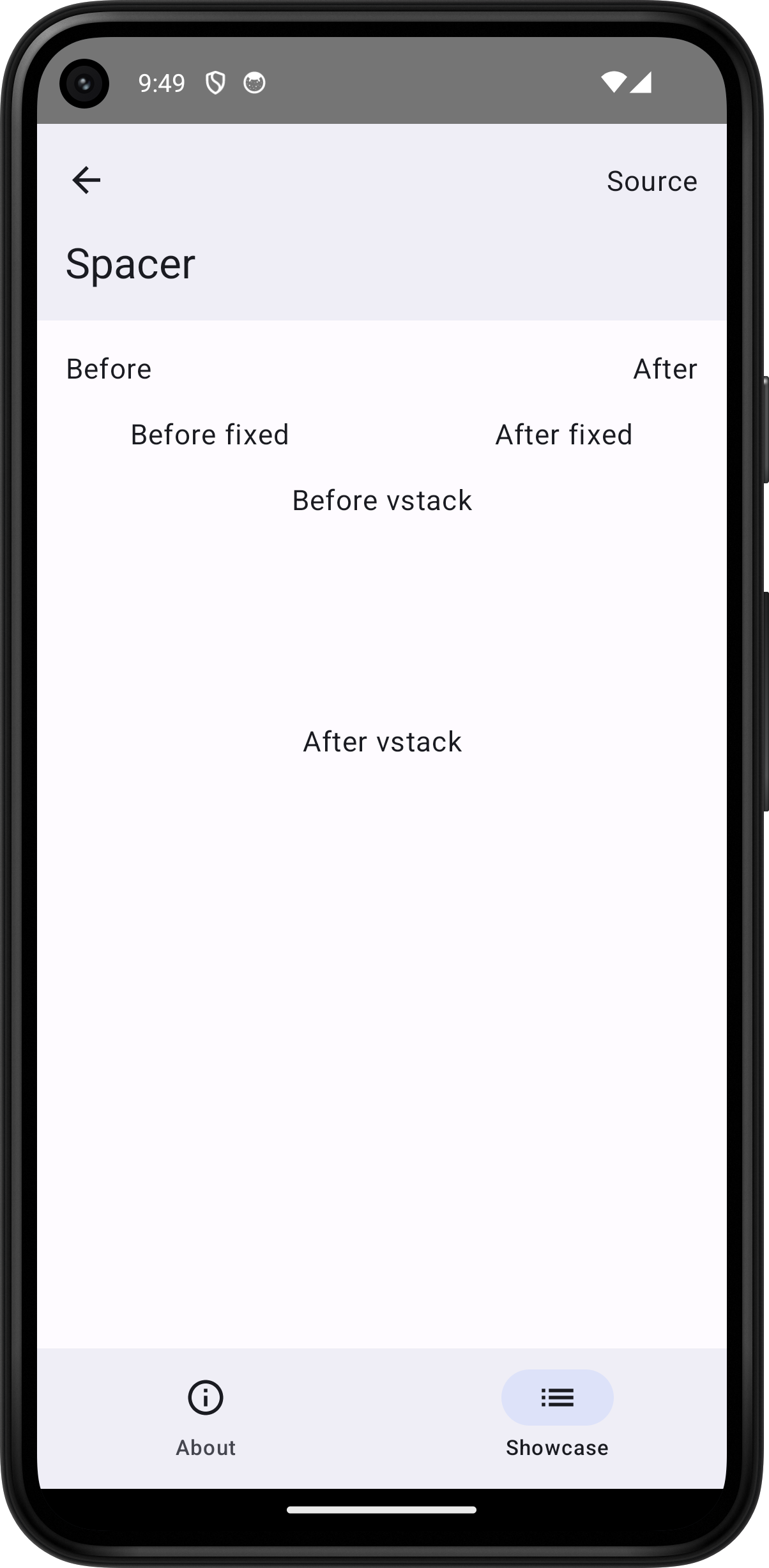The image is a detailed graphical representation of a smartphone mock-up, likely displaying an app interface design. The smartphone itself features rounded edges with a black border. At the top of the screen is a dark gray bar displaying icons for signal strength and Wi-Fi strength, along with the time reading 9:49. Additionally, there are two other unrecognized icons at the top. The front-facing camera is located in the upper left corner, suggesting it could be an Android device.

Beneath the dark gray bar, there's a light gray bar with the text "Source" and "Spacer," accompanied by a left-pointing arrow. The central portion of the screen is predominantly white or very light gray. On the upper left of this section, the word "Before" is displayed, while "After" is on the upper right. The subsequent line reads "Before Fixed" on the left and "After Fixed" on the right. Centered below these lines are the words "Before VStack" and, slightly lower, "After VStack."

At the bottom of the screen, there is another light-colored rectangle. This section contains a small circle button with a lowercase "i" accompanied by the label "About." Next to it is a hamburger menu icon with three lines, labeled "Showcase," which appears to be highlighted in the image. 

Overall, the mock-up provides a clear and structured view of the app's interface and layout elements.